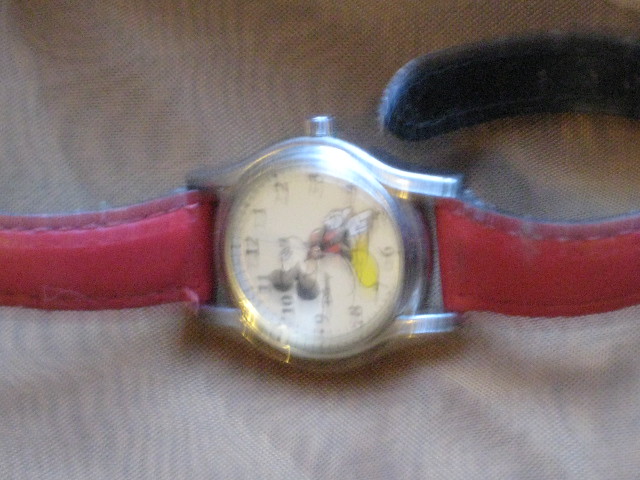A partially blurry photograph showcases a unique red wristwatch with a silver circular body at its center. Adorning the watch face is a charming image of Mickey Mouse, complete with his iconic black ears, white gloves, red shirt, and yellow shoes. The white watch face is marked with black numbers for easy readability, and some black text is visible near the number nine. Light reflects off the silver body of the watch, adding a subtle shine. The wrist strap, originally red, appears somewhat faded and frayed, indicating wear over time. The wristwatch is resting on a tan surface, adding a contrasting backdrop to the whimsical timepiece.